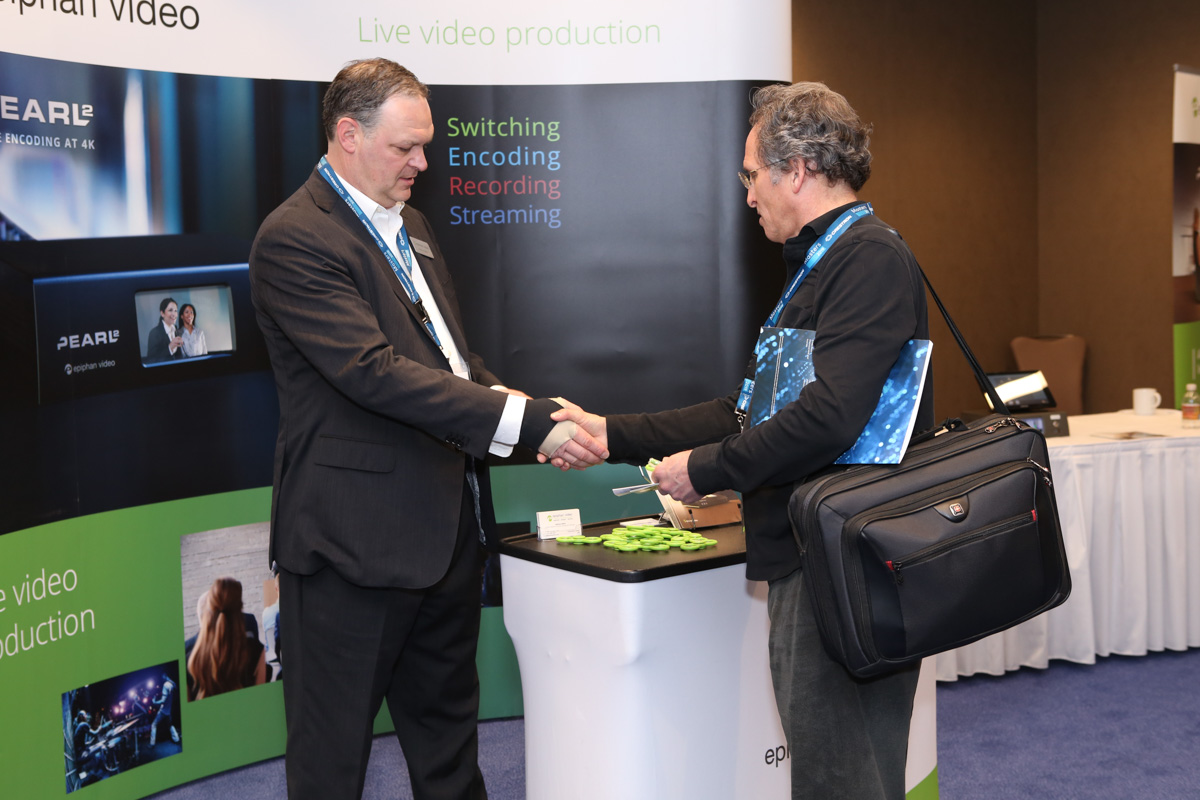This detailed, color photograph, taken indoors at a convention or event, captures two men shaking hands, prominently positioned in the center of the frame. The setting features dark blue carpeting and a backdrop of large banner displays advertising live video production services like switching, encoding, recording, and streaming in various colors. The man on the left, tall and wearing a black suit with a white shirt and a blue lanyard around his neck, has thinning hair. His right hand is extended in a handshake with the man on the right, who is slightly shorter, sporting a black turtleneck, gray slacks, glasses, and a similar blue lanyard. This man carries a large black bag over his shoulder and a blue notebook under his left arm. Both men are intently focused on their handshake. Behind them is a brown wall with a large screen or display, contributing to the convention atmosphere. Additional details include a white podium with a wooden top and green base situated in the foreground, and a table behind the men, adorned with a long white tablecloth, holding a coffee mug and water bottles. The banner behind the men has vivid text promoting various services and an image of two women accompanied by the text "Pearl" on the left-hand side.